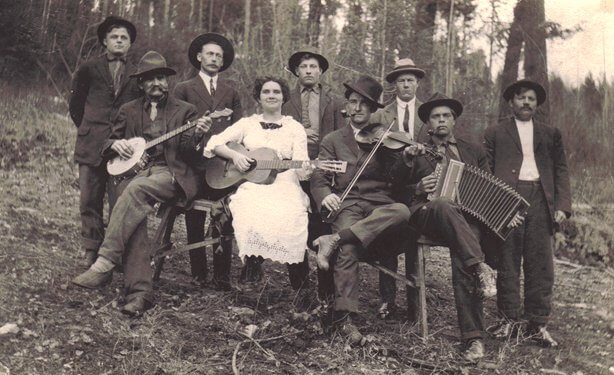This black-and-white photograph, likely from the 1920s, depicts a group of nine people posed outdoors in front of a wooded background with bare tree branches, suggesting it may be winter. The horizontally aligned rectangular image features eight men and one woman who are set in two rows, either standing or sitting on a wooden bench or possibly a picnic table. 

All the men are dressed in suits with collared shirts, and most are wearing ties and hats. On the far left, a man is seated with a banjo, flanked by two men standing behind him. At the center, the sole woman in the group sits in a chair, wearing a white dress and holding a guitar, smiling at the camera with her short brown hair. To her right, a man with a pipe in his mouth, wearing a hat, sits with his legs crossed while playing a violin or fiddle. Behind the woman is another man in a hat, staring directly at the camera without smiling. Further to the right, another man in the front row is sitting and playing an accordion, while two more men stand behind him. The ground beneath them is scattered with rocks, twigs, and branches, adding to the rustic, old-time feel of the photograph.